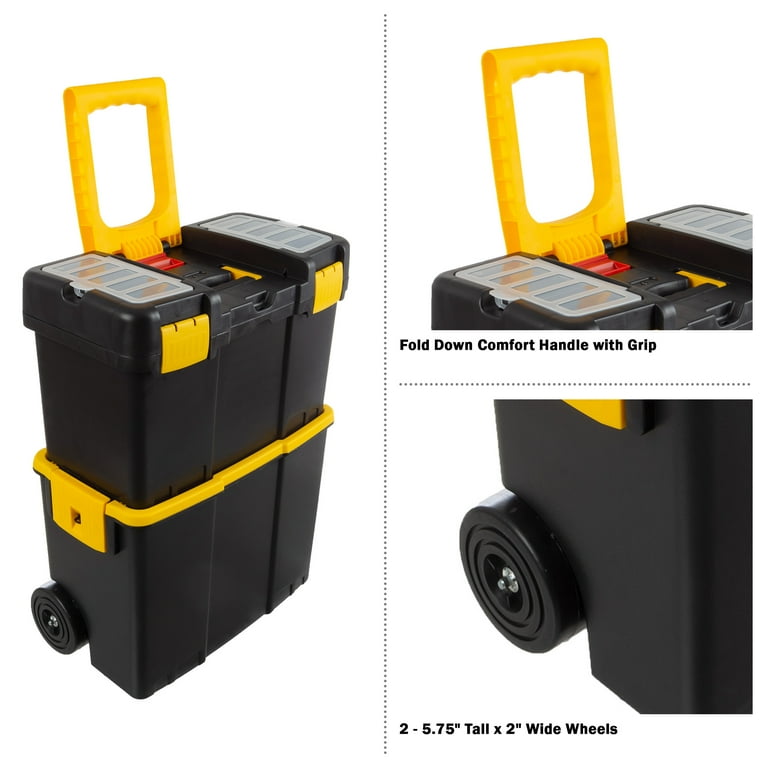The image depicts a black and yellow tool box on wheels, divided into two parts by a dotted line. The left side shows the complete tool box with a thick yellow handle on top, designed for easy wheeling. This portable storage unit consists of two stackable containers, secured by the yellow handle. The top container features two clear compartments for additional storage. The black wheels, which are 5.75 inches tall and 2 inches wide, make it convenient to move the box around. The right side of the image zooms in on specific components: the handle, which is described as a "fold-down comfort handle with grip," and the wheels, providing detailed dimensions. This tool box is ideal for transport and storage, likely used by professionals such as repairmen to carry tools to job sites.